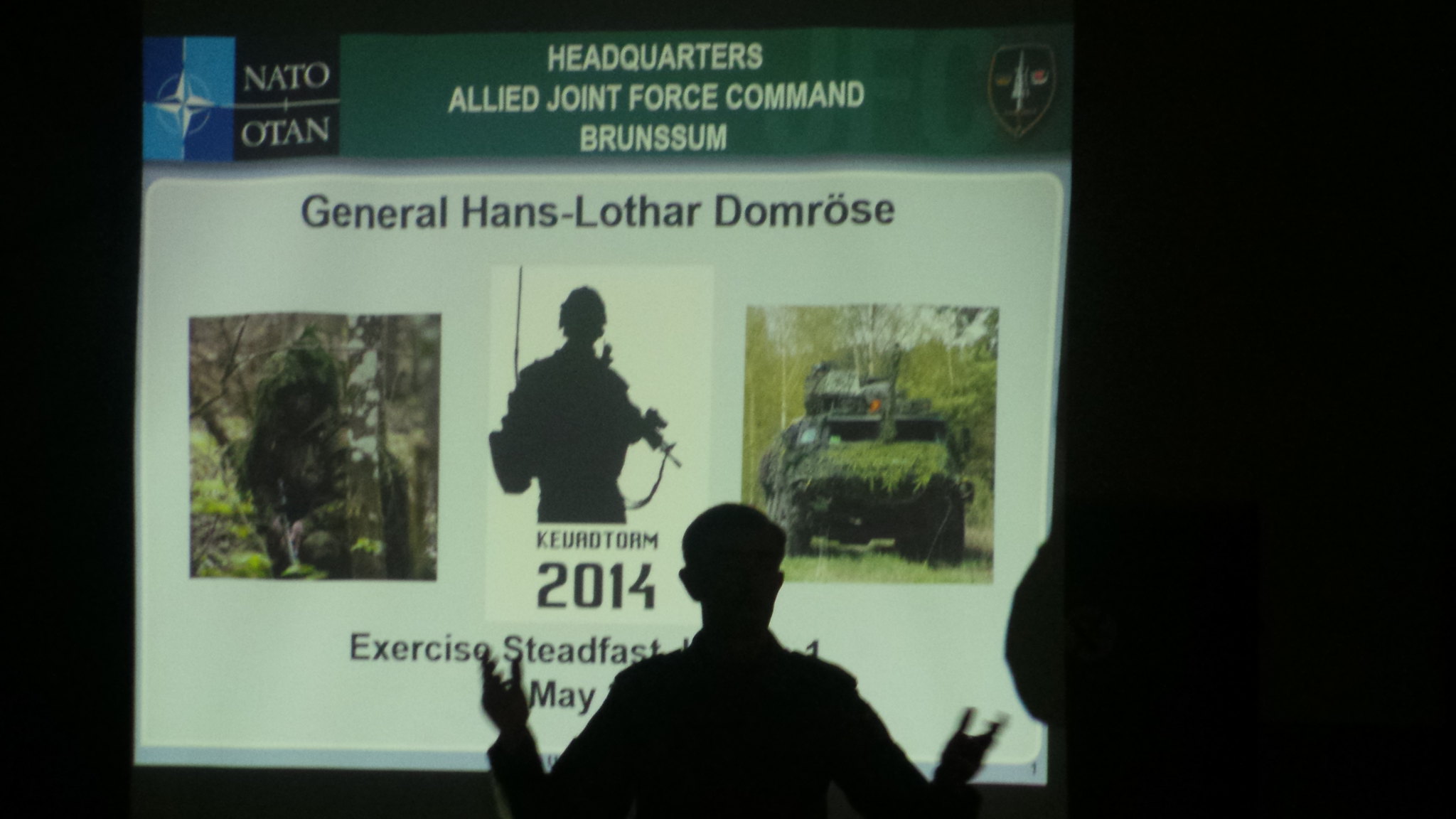This photograph, taken at a conference, features the silhouetted figure of a man addressing an audience, standing in front of a bright projection screen. His arms are outstretched with palms facing inward, emphasizing his engagement in the speech. The projection screen displays a banner with a green border at the top. In the upper left corner, it reads "NATO" followed by "O-T-A-N." The main header of the banner states, "Headquarters, Allied Joint Force Command, Brunssum." Beneath this text, it reads "General Hans Lothar Domros." The background is filled with imagery, including three distinct visuals: on the left, a soldier in full camouflage; in the center, an abstract silhouette of a soldier carrying a gun; and on the right, a color picture of a camouflage tank. The bottom portion of the screen, partially obscured by the silhouetted speaker, mentions "2014" and "exercise steadfast May." The image captures the commanding presence of the speaker against a backdrop rich with military references and insignia.